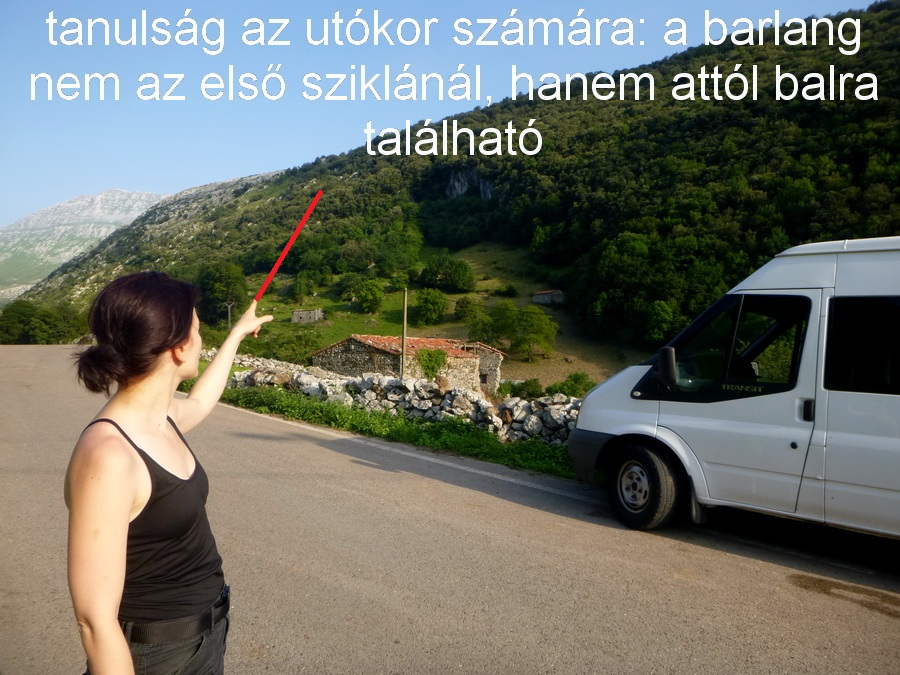A young Caucasian woman with brunette hair, pulled back slightly, is standing on the left side of the photograph near a country road with no traffic. She is wearing a black tank top, black jeans, and a black belt. Her left hand is extended, pointing towards a distant hill covered in green vegetation with shadows cast at the top right. From her pointing finger, a red line is superimposed on the image, reaching about three-quarters of the way up the hill, towards something difficult to discern. In the background, there's a cream-colored stone building with a red roof, situated at the base of the hill. Nearby, at the center of the image, is a utility pole, and there is a makeshift stone wall further ahead in the foreground. A white van with black trim is parked on the right side of the road, facing left. The photograph, taken on a sunny day, features three lines of white text in a foreign language at the top.